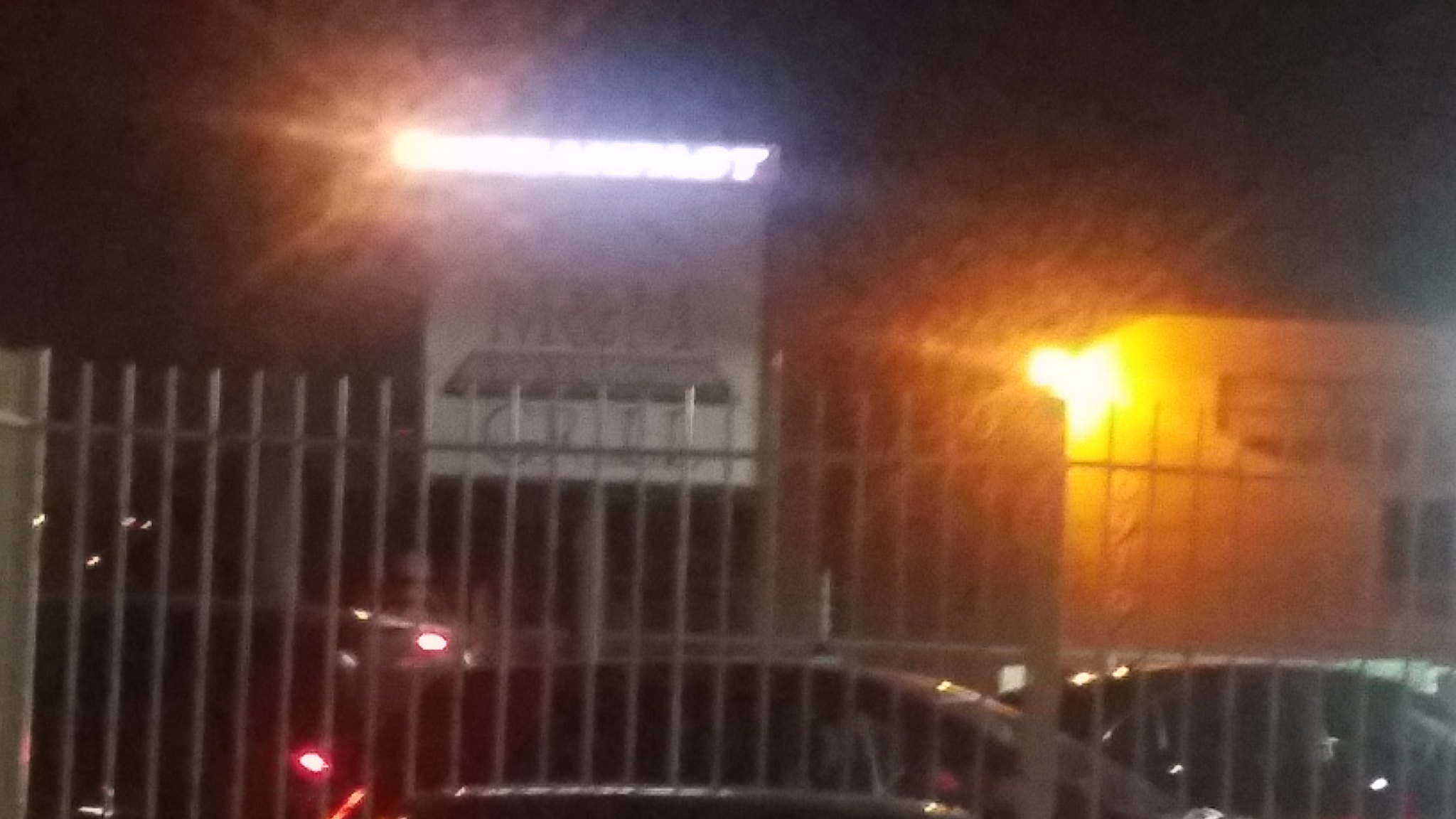The image depicts a blurry nighttime photograph, likely taken with dated technology, showcasing a fenced-off area that appears to be a private parking lot with some parked cars. The main focus is a metal gate with vertical bars positioned in front of a building. Behind the gate, there is a prominent square white sign encased in a house-shaped outline that reads "M&M Grill," although the text is hard to discern due to the image's poor quality. Above the sign is a light, along with another light to the sign's right, emitting a yellow-orange tone, possibly indicating the building is between other structures. Additionally, the blurred photograph features the number "0910" on the side of a building, enhancing the setting's atmospheric nighttime ambiance.